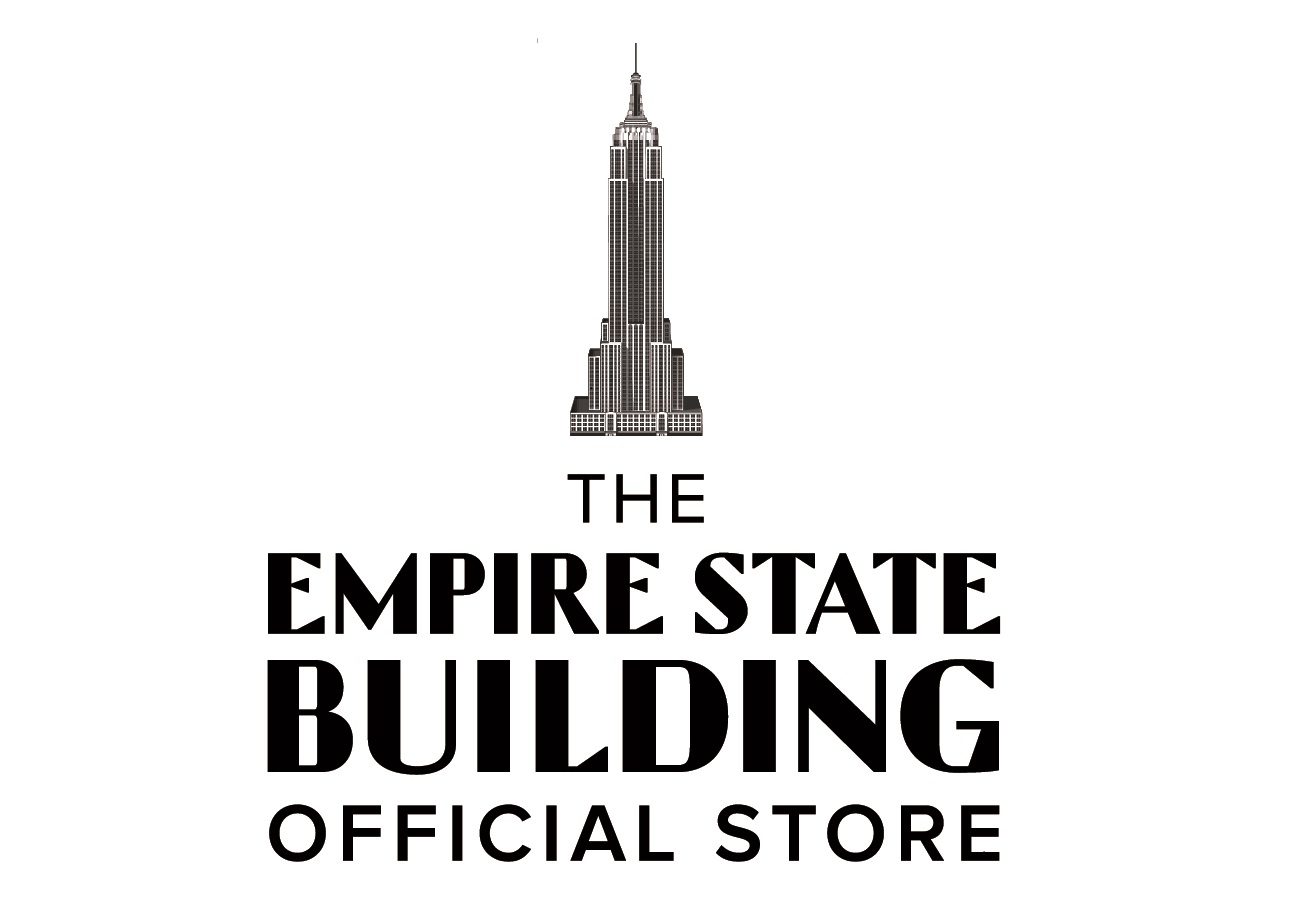The image is a sign advertising the official store of the Empire State Building. It features a white background with a mix of black text and a graphic. The top half showcases a stylized black outline of the iconic Empire State Building, depicted in line art that includes the building’s characteristic thick base and thin, towering top, culminating in a prominent antenna. This illustration has a somewhat logo-like format, with minimal detail emphasizing its tall, slender structure, and includes smaller buildings at its base, adding to the cityscape impression.

The bottom half of the sign contains four lines of large black text, arranged in a landscape orientation. The text reads: "The Empire State Building Official Store." "Empire State Building" is presented in a bold, retro-style font, contrasting with the block, all-caps "Official Store" below it.

Overall, the design maintains a black and white color scheme, combining elements of graphic design, typography, and illustration to effectively convey both the iconic image and the commercial purpose of the store.